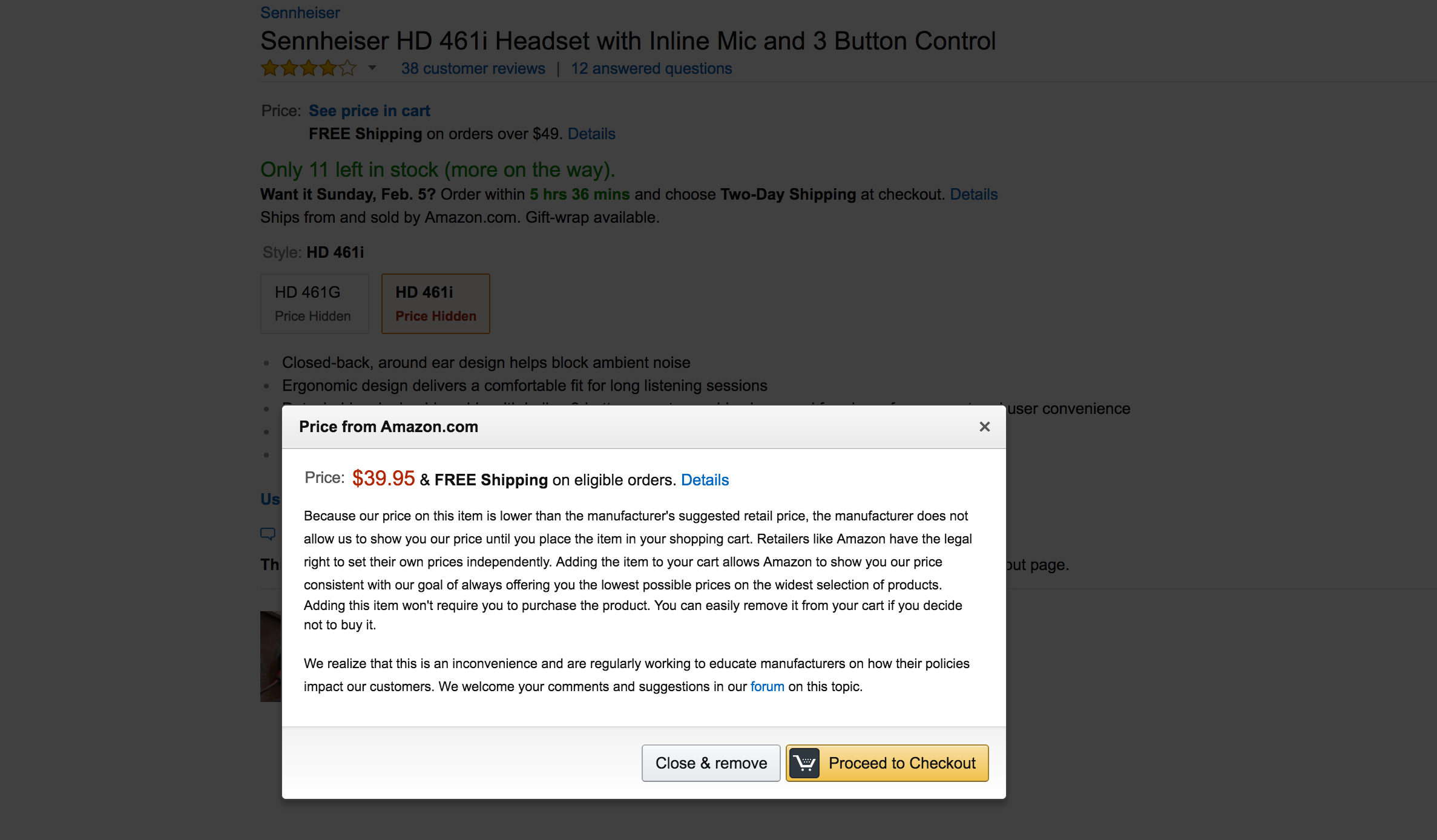The image is a screenshot of a section of the Amazon website displaying a special pricing notification. The open window within the screenshot states that the item has a price of $39.95 with free shipping on eligible orders. The text, highlighted in a light blue font, explains that because Amazon's price for this item is lower than the manufacturer’s suggested retail price, Amazon is not allowed to display the price until the item is added to the shopping cart. This policy is in place as retailers like Amazon hold the legal right to set their prices independently. Additionally, adding the item to the cart does not obligate a purchase, and it can be easily removed if the user decides not to buy it. The message acknowledges the inconvenience and mentions Amazon's ongoing efforts to educate manufacturers about the impact of their pricing policies on customers. The notification concludes with options to close the window, remove the item, or proceed to checkout.